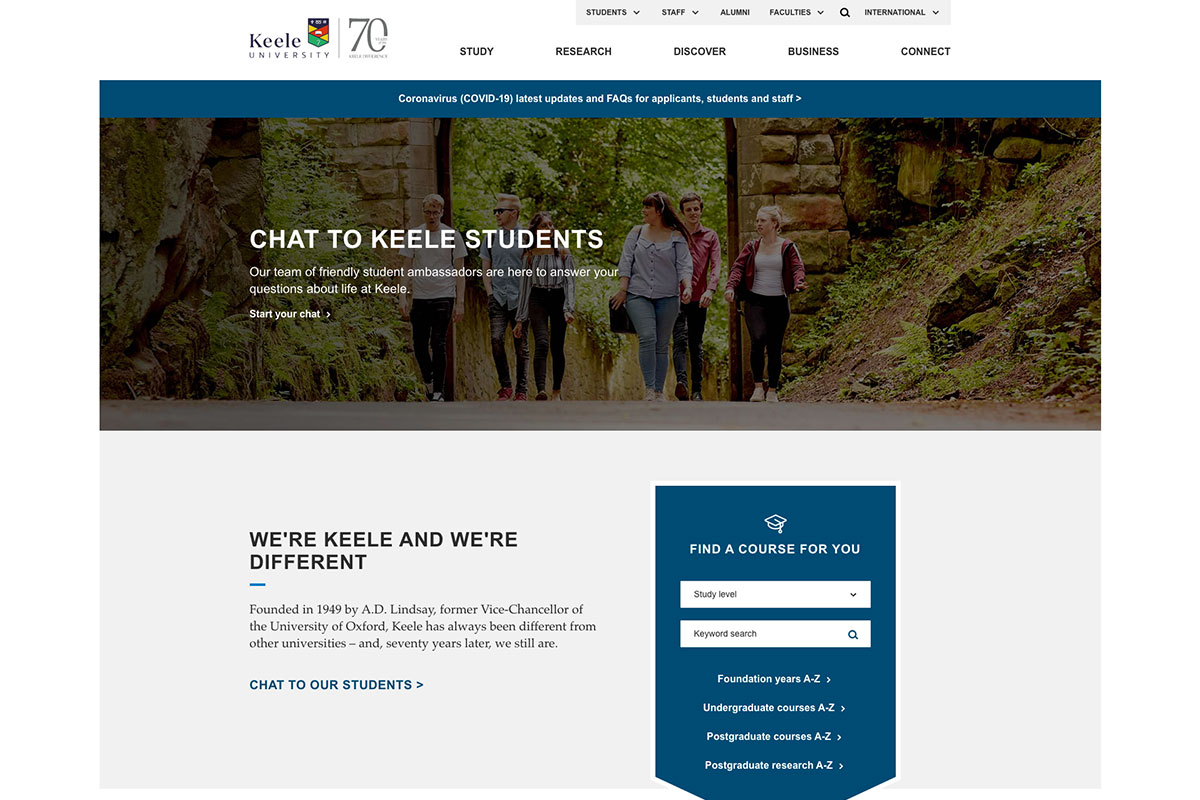This is a detailed, cleaned-up caption for the described image:

The screenshot is from the Keele University website, characterized by its clean white background with dark blue accents. The design includes a blend of black and blue text. Dominating the upper portion of the page is a panoramic banner photo depicting a group of six college-aged individuals—three men and three women—casually dressed in jeans and t-shirts. They are walking along a paved pathway with steep embankments composed of dirt, rocks, and green ferns on either side. A prominent brick archway in the background suggests they have just passed through it. The website's top section features the Keele University crest in the upper left corner, showcasing blue, yellow, red, and green colors, accompanied by navigation bars aligned to its right. Directly below the banner photo, which has the text "Chat to Keele Students," is a blue rectangular button inviting users to "Find a course for you," complete with search bars for further exploration.